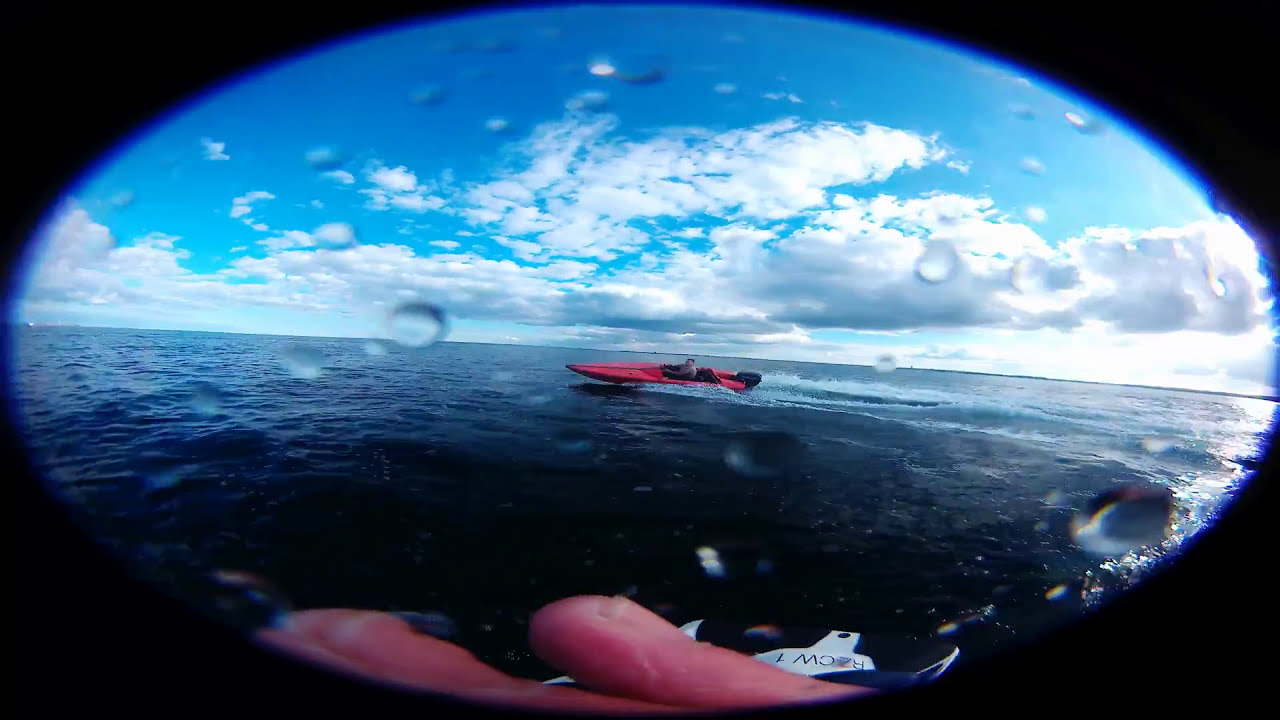Captured through a fisheye lens, this vivid photograph shows a high-speed adventure on a vast, open body of water. At the center of the image, a person is maneuvering a red and black motorboat, creating splashes that have left droplets on the camera lens, suggesting close proximity to the action. The motorboat appears to be moving quickly, possibly mid-turn, adding a dynamic sense of motion to the scene. In the foreground, two fingertips partially obscure the view, hinting that the picture was taken by someone on another vessel, possibly a jet ski or another boat. The overall image, slightly darkened around the oval-shaped edges due to the fisheye lens, contrasts with the bright and sunny day. The sky is a striking mix of large clouds and clear blue patches. In the distance, a few more boats are visible, as well as a hint of land, although the expansive water dominates the scene with its small, choppy waves.